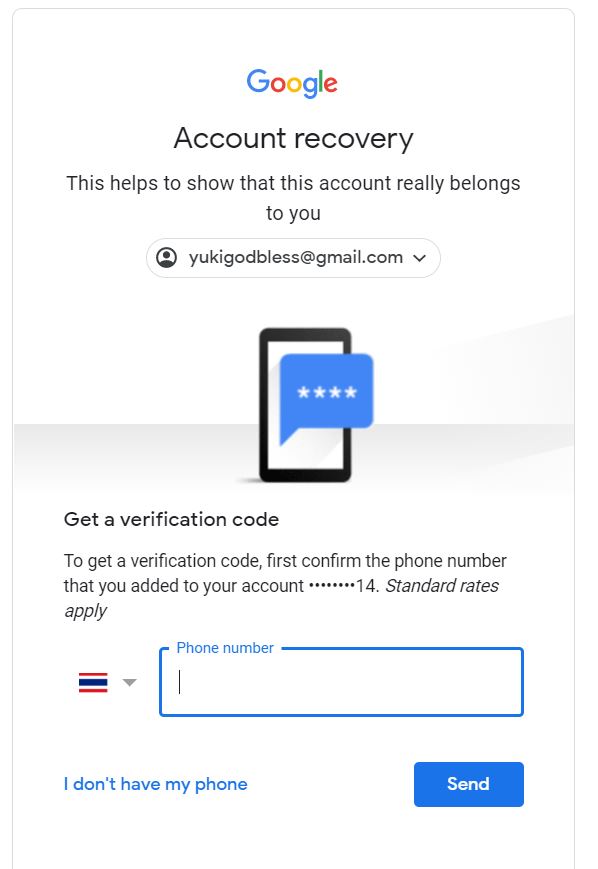The image consists of a user interface designed for Google Account Recovery. The layout begins with a gray-outlined rectangle featuring the word “Google” at the top, displayed in its signature multi-colored font. Below, it reads "Account Recovery" with a subheading stating, "This is to help show that this account really belongs to you."

Central to the image is a bulging rectangle with rounded sides, also outlined in gray, containing an icon of a person and an email address, accompanied by a downward-pointing arrow. Below this section, there is an illustration of a tablet, rendered in black and white, next to a blue speech bubble containing four stars.

Further down is a gradient box—shifting from light gray at the top to white at the bottom—with the instruction: "Get a verification code. To get a verification code, first confirm the phone number that you added to your account." This is followed by ellipses and the note “Standard rates apply.” Additionally, the section includes a symbol characterized by two thin red lines with a thicker blue line between them and another downward-pointing arrow.

To the bottom of the image, a blue-outlined rectangle is present, indicating a field for entering a phone number, followed by the option “I don’t have my phone,” and a blue rectangular button labeled “Send.”